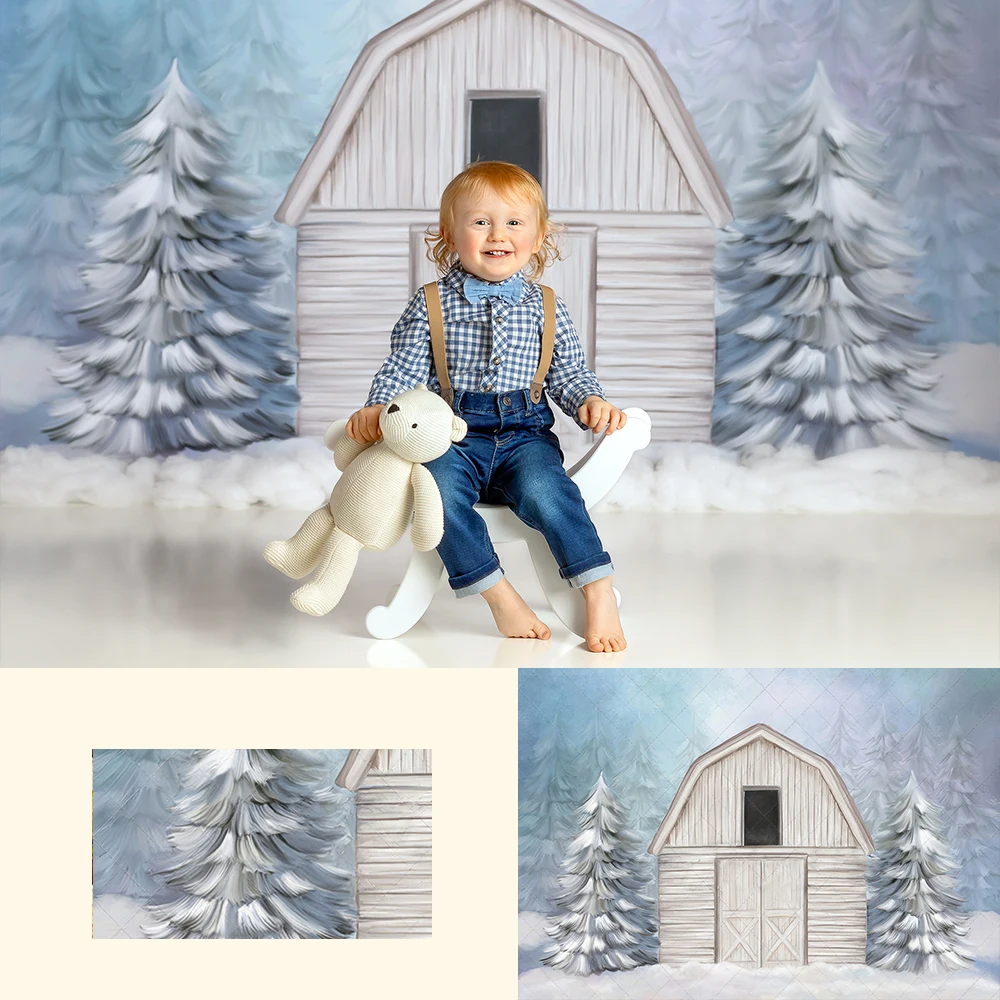A cheerful Christmas card photo captures a red-haired child with strawberry blonde curls sitting on a white bench in a festive winterscape. The child, adorned in a blue and white plaid shirt with a blue bow tie, brown suspenders, and rolled-up denim jeans, is barefoot with one foot folded underneath. He is happily clutching a simple white teddy bear, possibly a polar bear plushie. His radiant smile lights up the scene. The background features a painted barn-like structure surrounded by fake snow, enhancing the 3D effect. Two tall pine trees flank the barn, with additional trees faintly visible further back, contributing to the wintry ambiance.